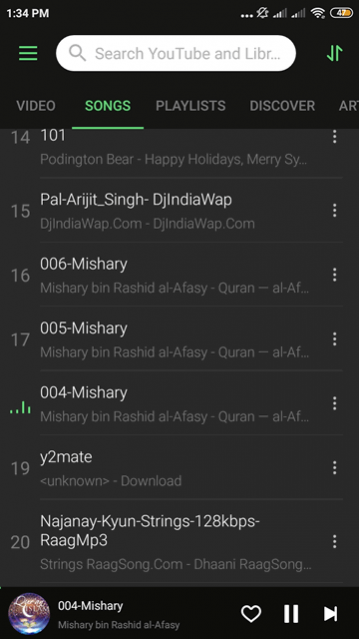The screenshot depicts a cell phone interface within the YouTube app, showcasing a playlist of songs. At the very top of the image is a black horizontal bar displaying the phone's status. On the left, it shows the current time, 1:34 PM, while on the right, icons indicate the phone's data and signal strength along with the battery life at 47%.

Below the status bar is a white horizontal bar featuring a search box labeled "Search YouTube and library," allowing users to search both YouTube and their device's media library. Underneath this, a horizontal menu offers tabs labeled "Videos," "Songs," "Playlists," and "Discover." The "Songs" tab is highlighted in green, signifying it as the active section.

The main content of the screen is a vertical list of songs numbered 14 through 20, appearing to be in Arabic or another Middle Eastern language. These tracks can be played by tapping on their respective links. The song in position 18 is currently playing, indicated by a green music bar in place of the number.

At the bottom of the screen, specific details about the currently playing song (number 18) are visible. This section includes the album art on the left and the song's name, title, and description centered at the bottom.